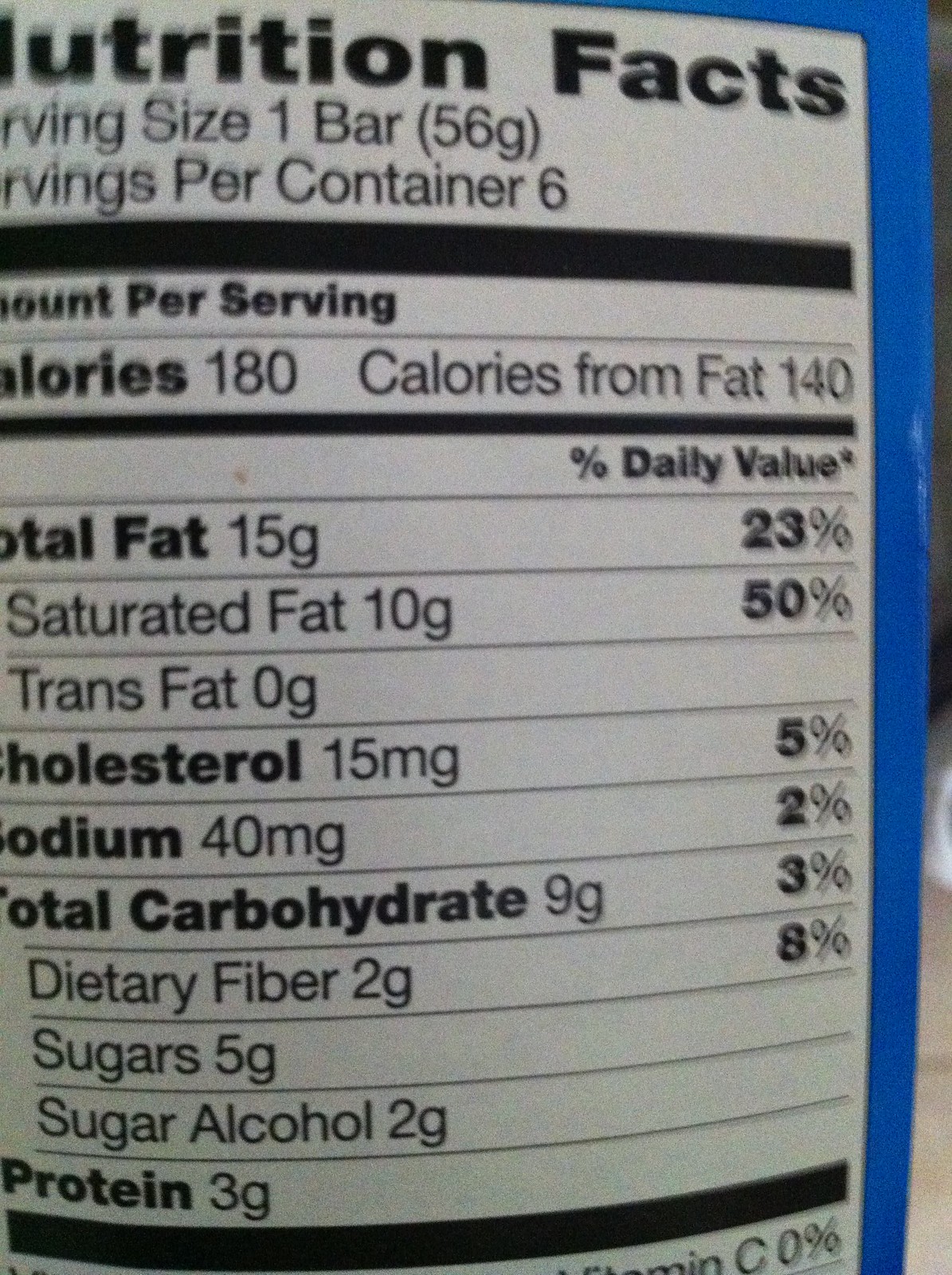This color photograph, shot in portrait mode, is a close-up of a nutrition label on a food package set against a bright blue background. The label, occupying the majority of the image, is rectangular with a white backdrop and black text. At the very top, it prominently states "Nutrition Facts." Key details on the label include: serving size of 1 bar (56 grams), with 6 servings per container. Each serving contains 180 calories, with 140 calories from fat. Nutritional components are detailed as follows: 15 grams of total fat (23% daily value), 10 grams of saturated fat (50% daily value), 0 grams of trans fat, 15 milligrams of cholesterol (5% daily value), 40 milligrams of sodium (2% daily value), 9 grams of total carbohydrates (3% daily value), 2 grams of dietary fiber (8% daily value), 5 grams of sugars, 2 grams of sugar alcohol, and 3 grams of protein. The photo also narrowly shows part of a tabletop in the extreme right background, yet the type of food remains unidentified as the front of the package is not visible.